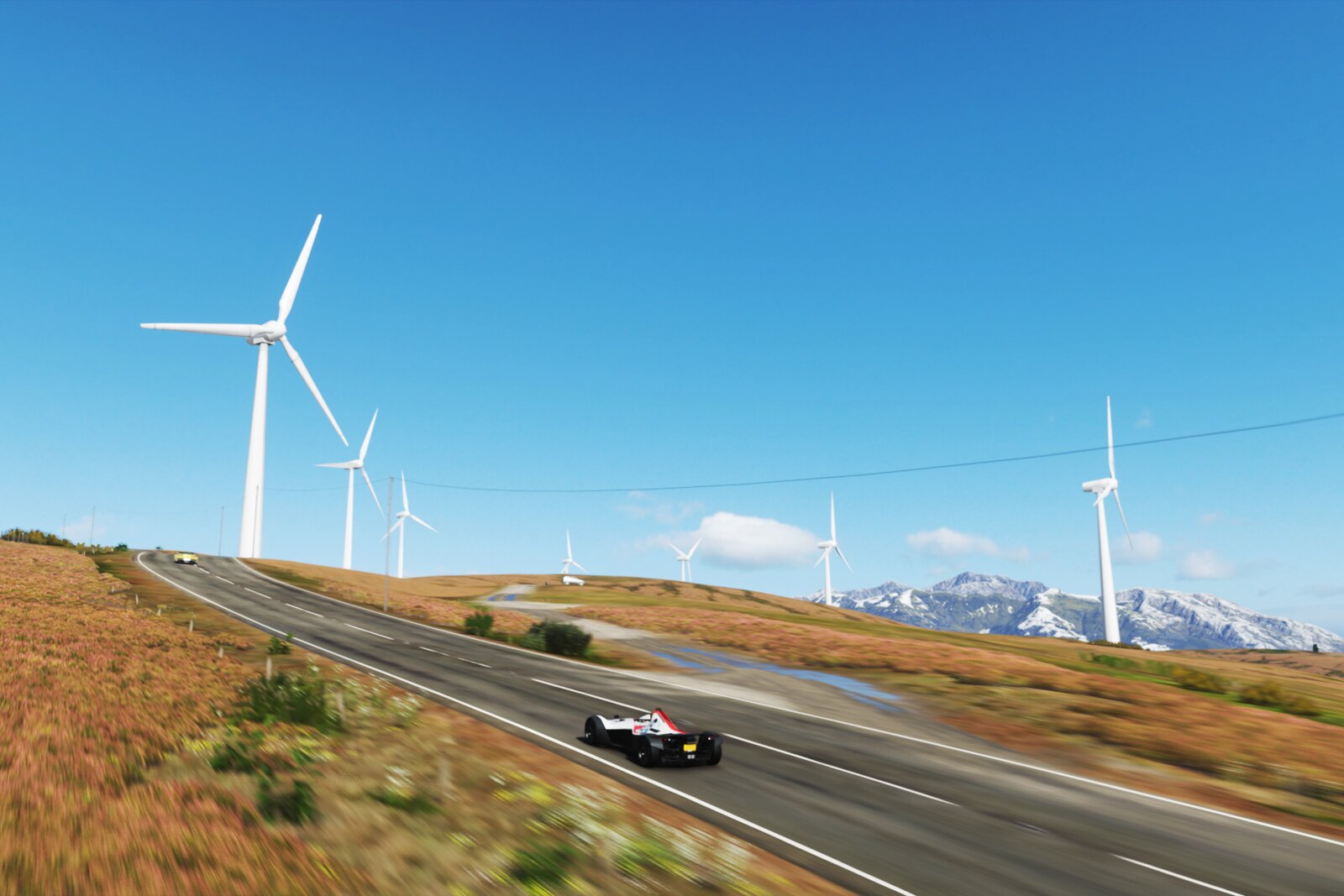This captivating image captures a sleek and sporty F1 car, vividly painted in white, red, and black, speeding along a well-kept two-lane road. The motion blur effect enhances the sensation of high speed, suggesting the car is moving exceedingly fast, possibly beyond the speed limit, adding an edgy feel to the scene. In the distance, another race car, possibly yellow, can be seen, contributing to the dynamic racing atmosphere. The road winds through picturesque plains and undulating hills, dotted with patches of green and brown vegetation. Numerous wind turbines, around seven, are scattered across these open fields, harnessing the wind under a clear, bright blue sky with a few low-lying clouds. The majestic, snow-capped mountains tower in the background, completing this photorealistic depiction of nature converging with high-octane motorsport.